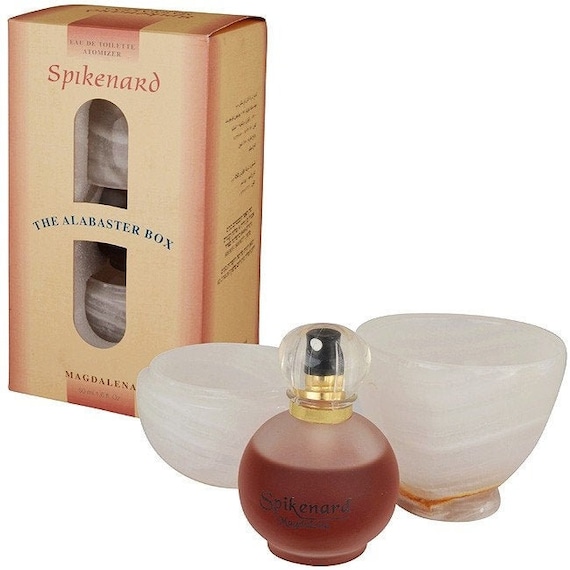This image depicts a vintage product display featuring a yellow-tinted cardboard box with a gradient orange border labeled "Aladé Toilette Atomizer" at the top center, and "Spikenard" beneath it in red text. This box has two semi-oval cutouts showcasing foam-held pieces, framing the text "The Alabaster Box," written in a blue, curved Times New Roman font. At the bottom of the box, the text "Magdalena" is visible. 

To the right of the box are two frosty, smoky whitish-colored stone bowls; one shorter and rounder, the other slightly taller and more oval. In front of these bowls is a spherical glass perfume bottle with a smoky, slightly red-tinted base containing a dark amber or reddish rosé liquid. The bottle is equipped with a black spray pump covered by a clear plastic cap. This meticulous arrangement emphasizes the elegant and vintage aesthetic of the spikenard perfume and its accompanying accessories.